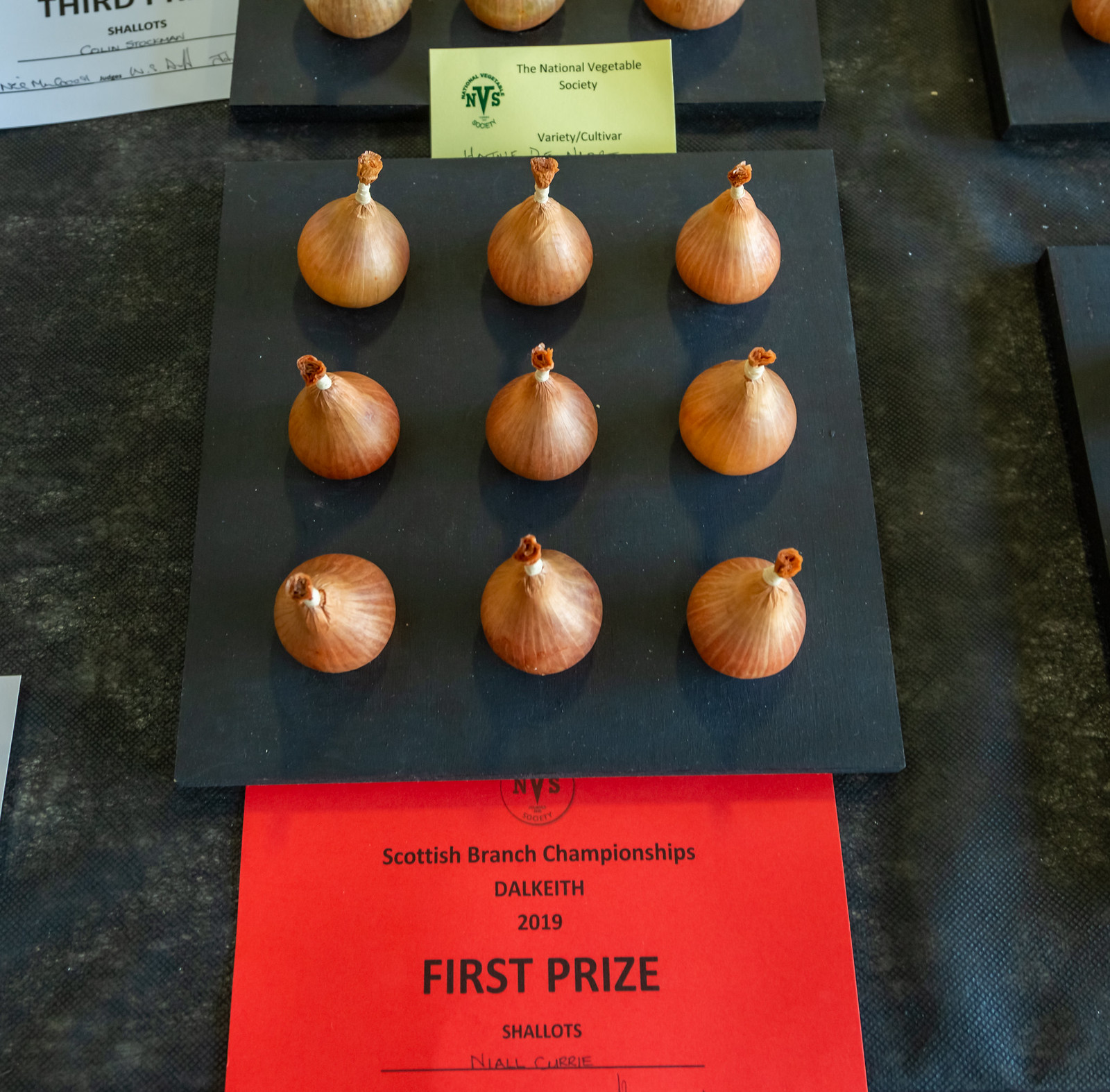The image depicts a meticulously arranged display of nine shallots, mistaken by some for onions or even Hershey's Kisses due to their appearance and copper-like color. These shallots are neatly organized in a three-by-three grid on a black surface. At the top of the display, a yellow card bearing the inscription "National Vegetable Society" is visible, indicating the association behind the contest. At the bottom of the arrangement, a red card with black writing reads "Scottish Branch Championships, Dalkeith 2019, First Prize, Shallots," with "Niall Currie" handwritten as the winner. The image showcases Niall Currie's first prize-winning entry in the shallots category at a prestigious vegetable competition.